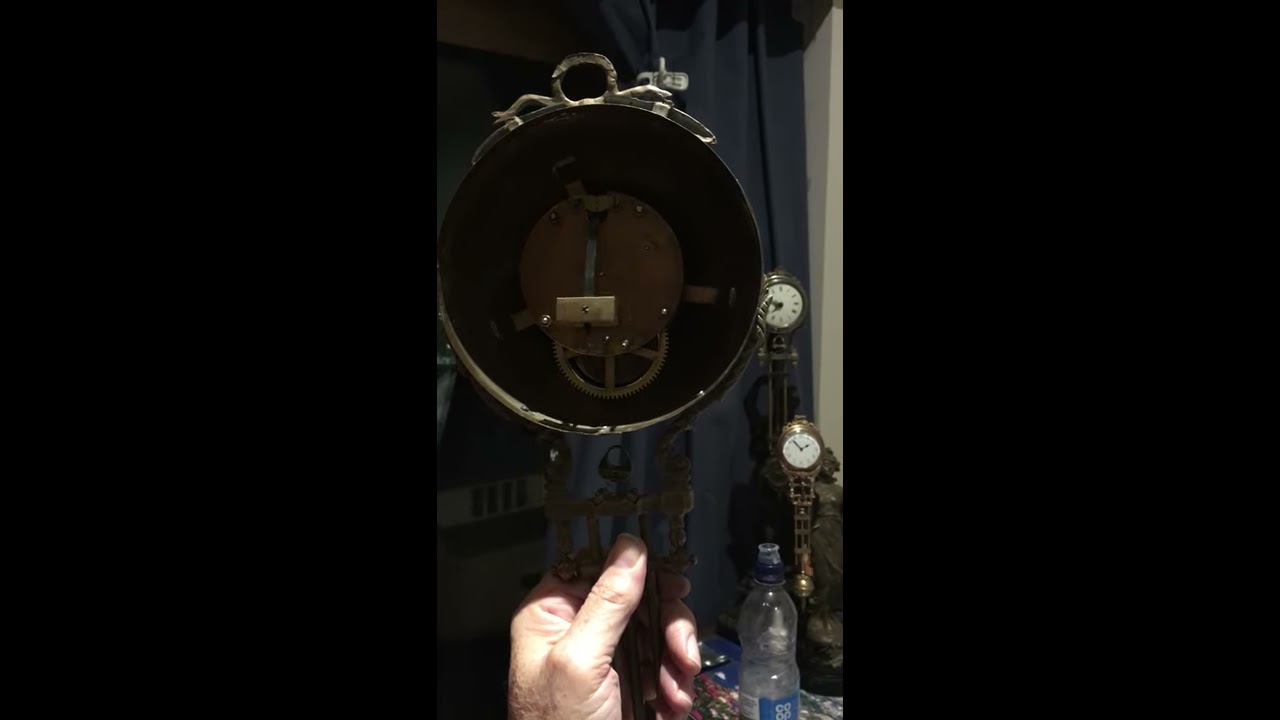In the photograph, a person's left hand is holding a small, circular brass clock that is missing its face, revealing its intricate gears and inner mechanisms. The image, captured vertically on a camera phone and framed by large black boxes on either side, emphasizes the clock's hollow, deconstructed state. Behind the hand, there are two complete clocks in a similar brass style, displaying their faces, with one showing two o'clock. Additionally, a blue robe hangs in the background, adding a touch of color. A water bottle is also positioned to the side of the held clock, further enriching the scene's detail.